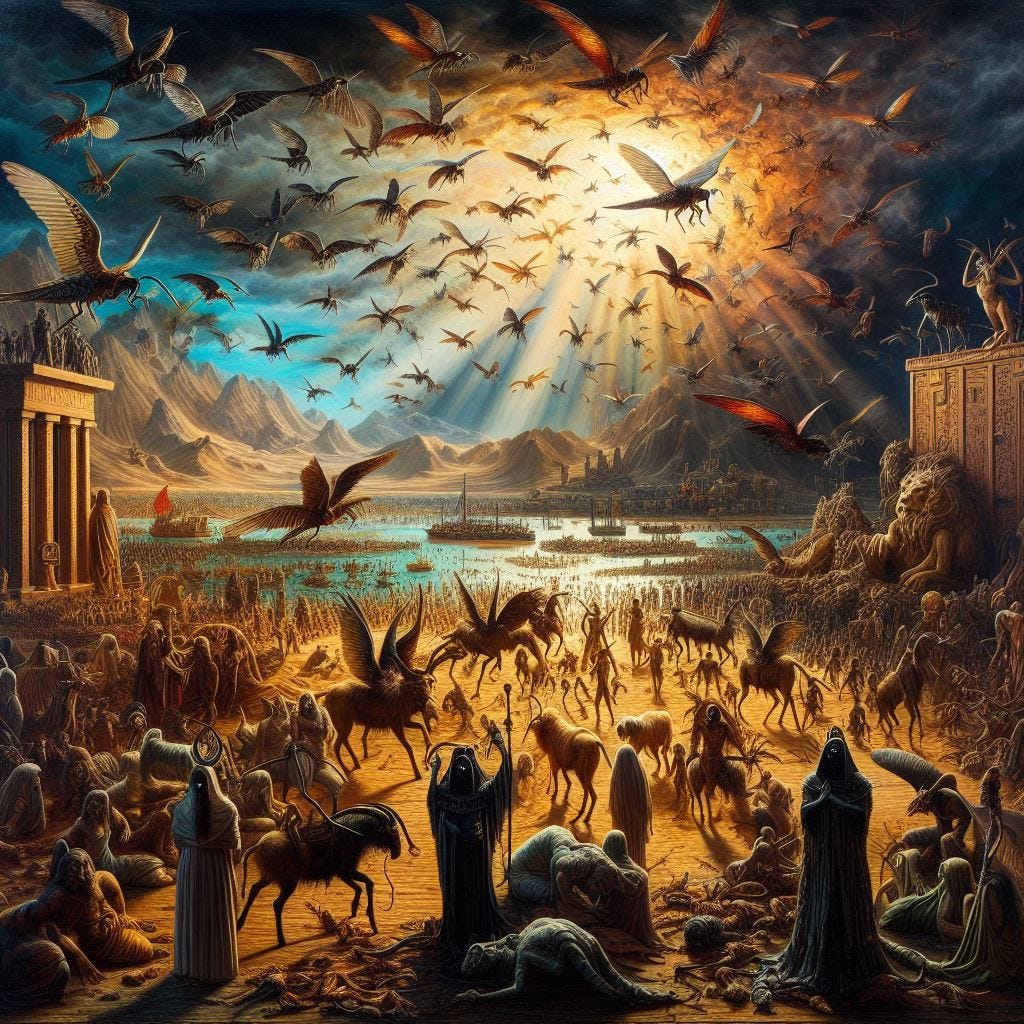This intricate and richly detailed painting depicts a surreal medieval scene teeming with activity. In the background, looming mountains and a serene lake are barely visible under a sky swarmed with hundreds of giant, winged insects, casting an almost apocalyptic shadow over the entire landscape. The once clear sky, only showing hints of blue near the horizon, is dominated by dark clouds and the blazing sun trying to pierce through. Among the chaotic aerial scene, a dragon can be faintly discerned.

On the land below, a myriad of mythical creatures and artistic sculptures, including imposing stone lions, add to the complex tapestry. The ground is sporadically dotted with hooded and robed figures, possibly in prayer, evoking a sense of mysticism. These figures are surrounded by various fantastical beasts, some with wings, adding to the eerie ambiance. Temple-like buildings adorned with additional sculptures stand tall, further contributing to the scene's medieval and otherworldly atmosphere.

In the distance, there are several ships, notably one with a red sail, suggesting a narrative of exploration or escape. The painting is a spectrum of vibrant and muted colors, featuring shades of grey, blue, yellow, black, red, brown, and orange. There is no text within the image, reinforcing its mysterious and surreal nature. The entire scene is rendered in a style that evokes classical medieval artistry, making the viewer feel as if they are peering into an ancient, fantastical world.